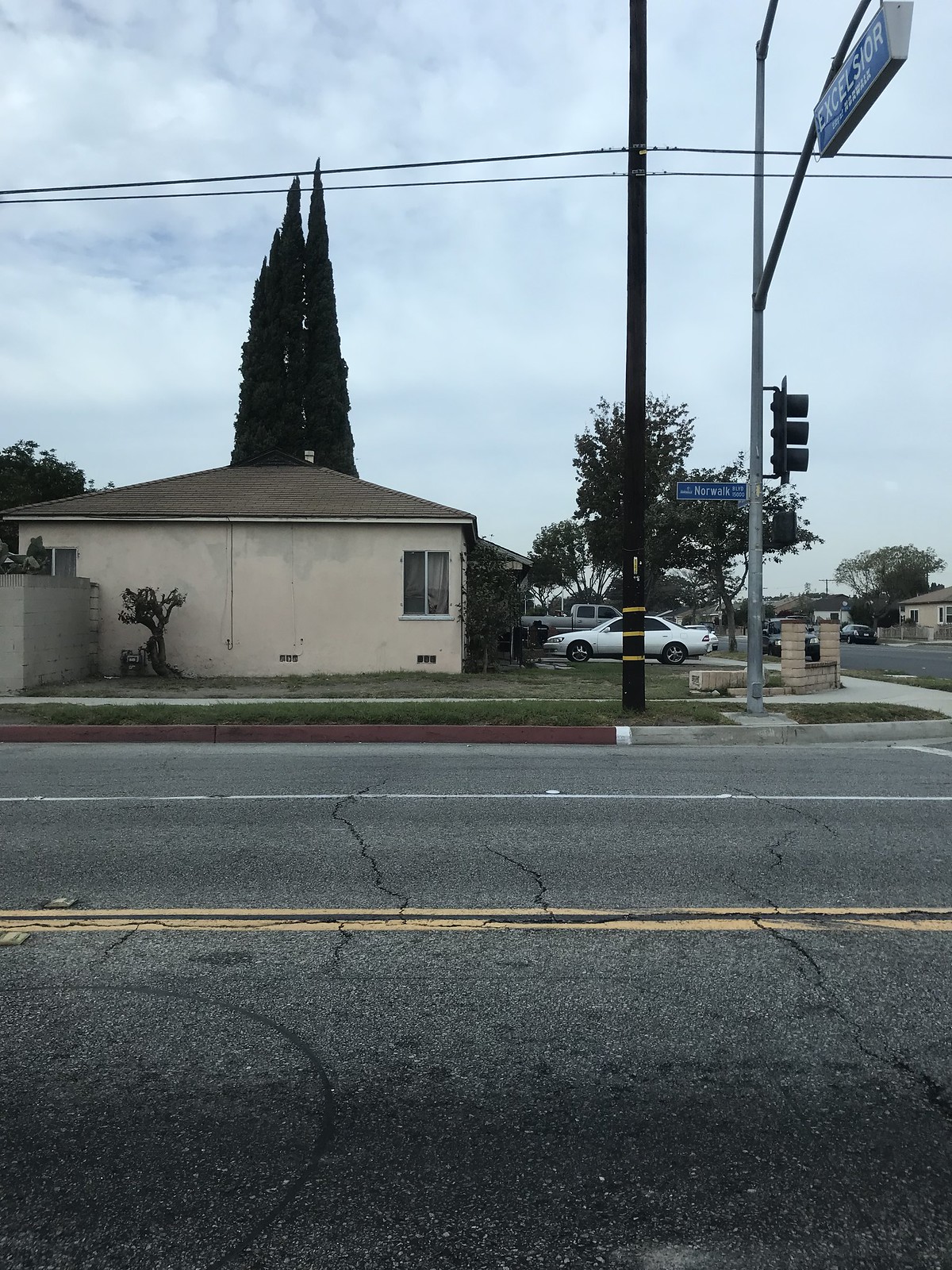The photograph captures a street corner view of a single-story home situated at the intersection of two streets. The asphalt road in the foreground appears significantly worn, riddled with numerous cracks and flanked by a faded double yellow line. Across the street from the home, a white stripe is painted on the curb, followed by a long stretch of dark brown pavement leading to a perpendicular sidewalk.

The home itself is constructed from stucco and exhibits signs of water damage on the visible side. A sliding window occupies a section of the wall. Planted close to the home is a small, short tree, while the front yard features a scattering of bushes and small trees lining one side of the front door. The driveway hosts a white or silver sedan, contrasting against the dry, sparse grass that looks particularly unhealthy.

In the vicinity, there's a green or blue street sign with white lettering mounted on a light pole and a traffic light visible from the side. A wooden utility pole, bearing electrical and telephone wires, stands nearby. Dominating the background on the far side of the home are two very tall pine trees with pointed tops, adding a touch of verticality to the suburban scene.